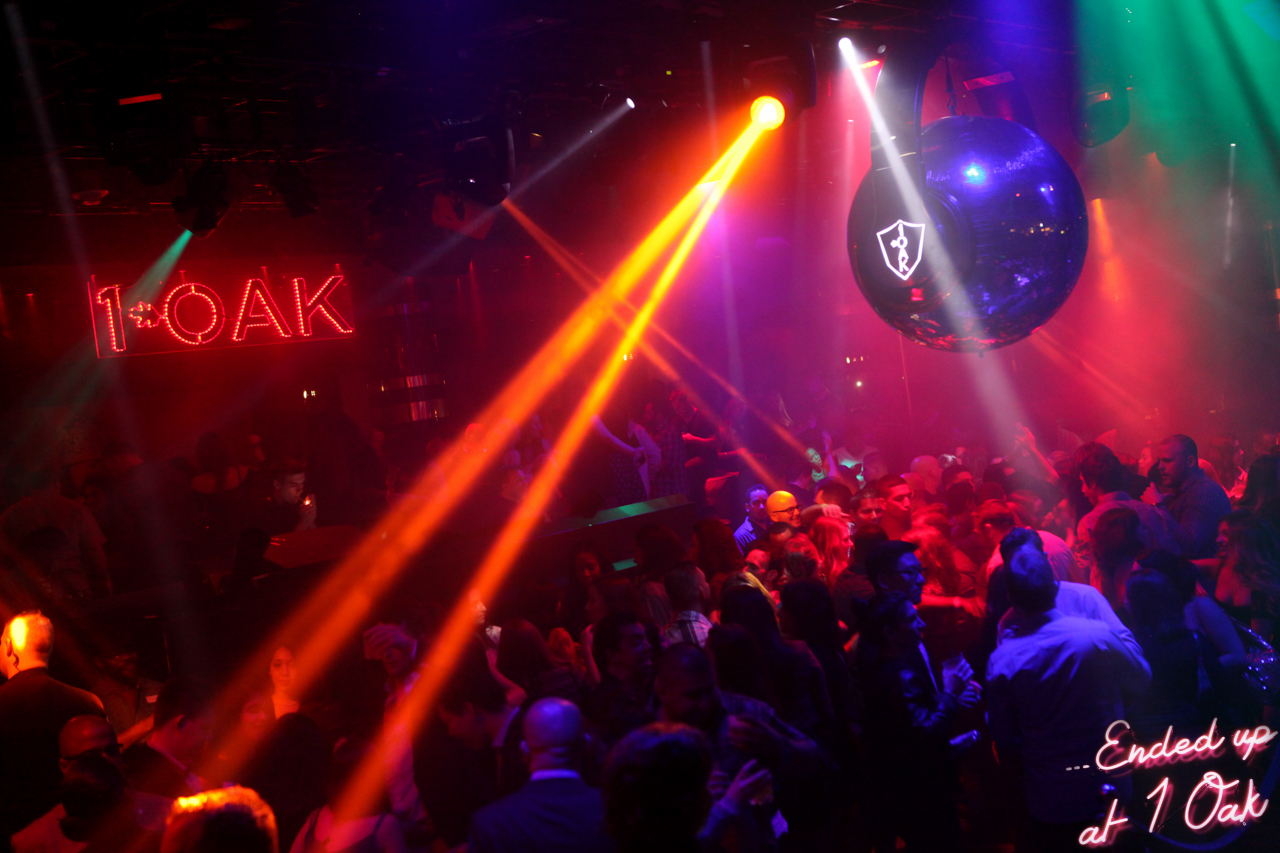The image presents a bustling scene inside a dark club packed with hundreds of people on the dance floor, dancing, socializing, and enjoying the music. A large, distinctive crystal ball hangs prominently from the ceiling in the upper right corner, secured by an arch that somewhat resembles a pair of headphones. Below this ball, which features a badge symbol with light white letters, blue light reflects off it, adding to the colorful ambiance. The upper right corner of the room also features contrasting green and brown curtains. Overhead, spotlights cast beams of light in various hues, including bright orange and white, illuminating different sections of the crowd. The white spotlight shines on the bottom right, while the orange spotlight creates a unique splitting pattern as it reaches the lower left. 

The lighting further complements the room's dynamic atmosphere, painting the crowd in vivid colors—people in the upper right are bathed in a red tint, while those in front of them are tinged with blue. Meanwhile, the far left side of the crowd is shrouded in shadows. Adding to the club's aesthetics, a fluorescent light on the left displays "1 O-A-K" in red neon letters. Another feature is the cursive white "Ended up at One Oak" message in the lower right corner, accented by a subtle red shadow. Amidst the throng, a figure can be seen in the background lighting a cigarette, contributing further to the vibrant and energetic environment of the club.